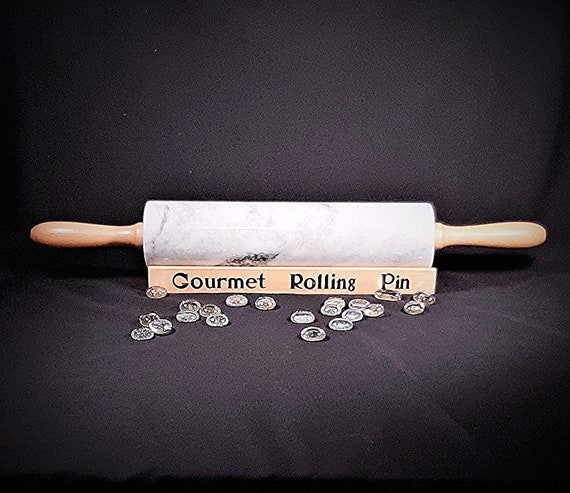In this low-resolution product photograph, likely intended for culinary enthusiasts or an advertisement, a detailed and sophisticated gourmet rolling pin is prominently displayed. The centerpiece of the image is the rolling pin, placed centrally, with its handles extending from left to right. The handles are crafted from a warm, tannish wood, contrasting elegantly with the rolling pin's cylindrical middle section, which boasts a glossy marble finish in shades of white and light black.

The rolling pin rests securely on a matching wooden base designed to prevent it from rolling—this base bears the black text “Gourmet Rolling Pin.” The backdrop is composed of a dark gray or black fabric that provides a stark contrast to the pin’s lighter colors. Scattered in front of the base are small, clear, glass beads, adding an intricate and decorative element to the setting. This rolling pin, with its luxurious appearance and functional design, is clearly aimed at gourmet cooks who appreciate both practicality and aesthetics in their kitchen tools.